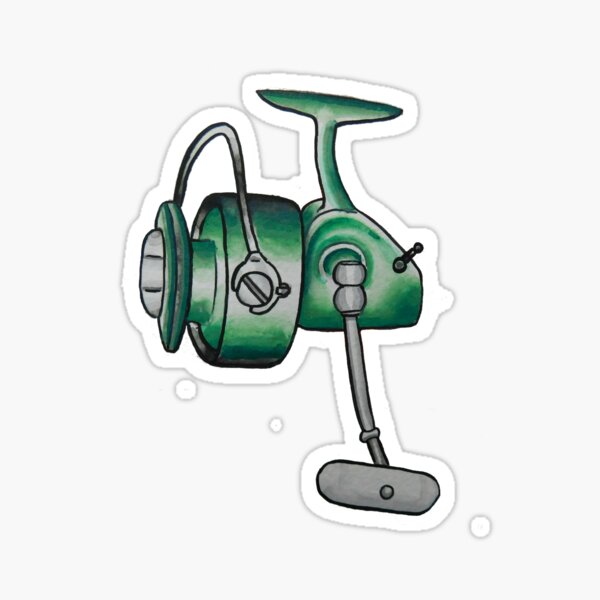The image is a detailed cartoon digital drawing featuring a green cylindrical machine that resembles a motor or a piece of equipment, potentially a weed whacker or lawnmower component. The device is marked by a prominent flathead screw on the left side, which secures a grounding wire, indicating it's part of an electrical apparatus. The cylindrical section on the left has a circular or cylindrical object, possibly an exhaust fan, and an extended bar making a T-shape that might serve as a handle. Attached to this cylindrical part is another green structure resembling a gas tank, from which a thin pole extends upward and splits into a T-shape. On the right side of this gas-tank-like object is a small metal lever, and below it, an arm extends outward and down, suggested to look like a professional microphone stand. The entire contraption is encompassed by a white bubble border, contributing to its sticker-like appearance, set against a plain white background. The image combines elements that evoke various interpretations, from mechanical motors to a meat grinder, illustrating intricate details such as the grounding wire and screws, accentuating its animated and meticulously designed nature.